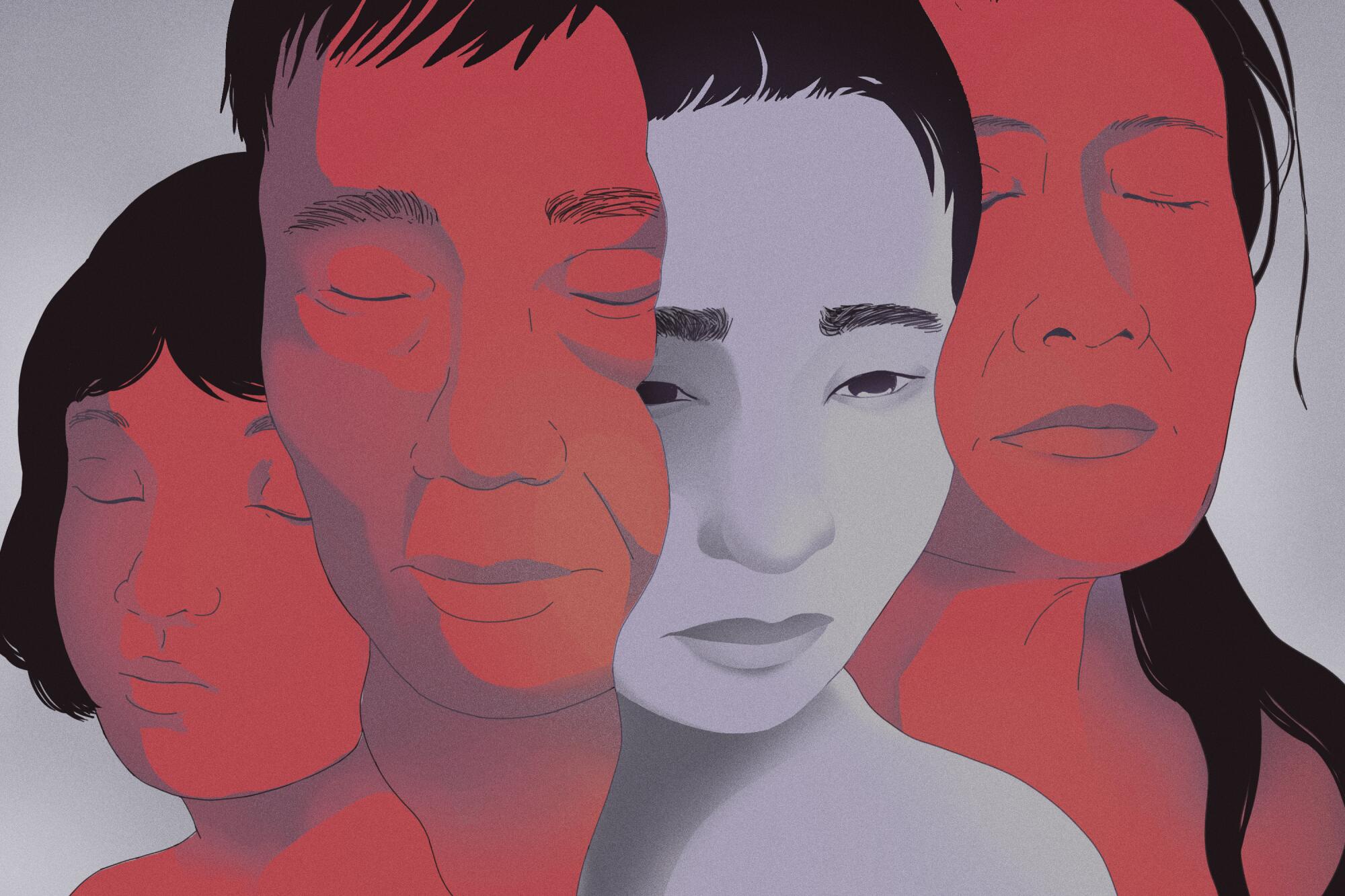This illustration depicts an emotionally evocative scene featuring four individuals against a gray background. From left to right, the first character is a young girl with short, dark hair parted in the middle. Her eyes and mouth are closed, and she has a reddish complexion. Next to her is a man with short, dark hair and a featureless, closed mouth. His eyes are also closed, and he shares the same reddish hue. The third individual is a gray-toned woman with a light purple tinge. Her black hair flows around her melancholic face, and she gazes downward with a somber expression. Finally, on the far right, there is another woman with long black hair, closed eyes, and a closed mouth; she too has a reddish complexion. All four figures appear to be closely connected, with the gray woman squeezed between the two reddish-hued parents, suggesting familial ties. The figures look almost nude, blending into one another, creating a sense of unity and shared sorrow. The entire image is sketched, capturing a poignant moment that reflects deep sadness and introspection.